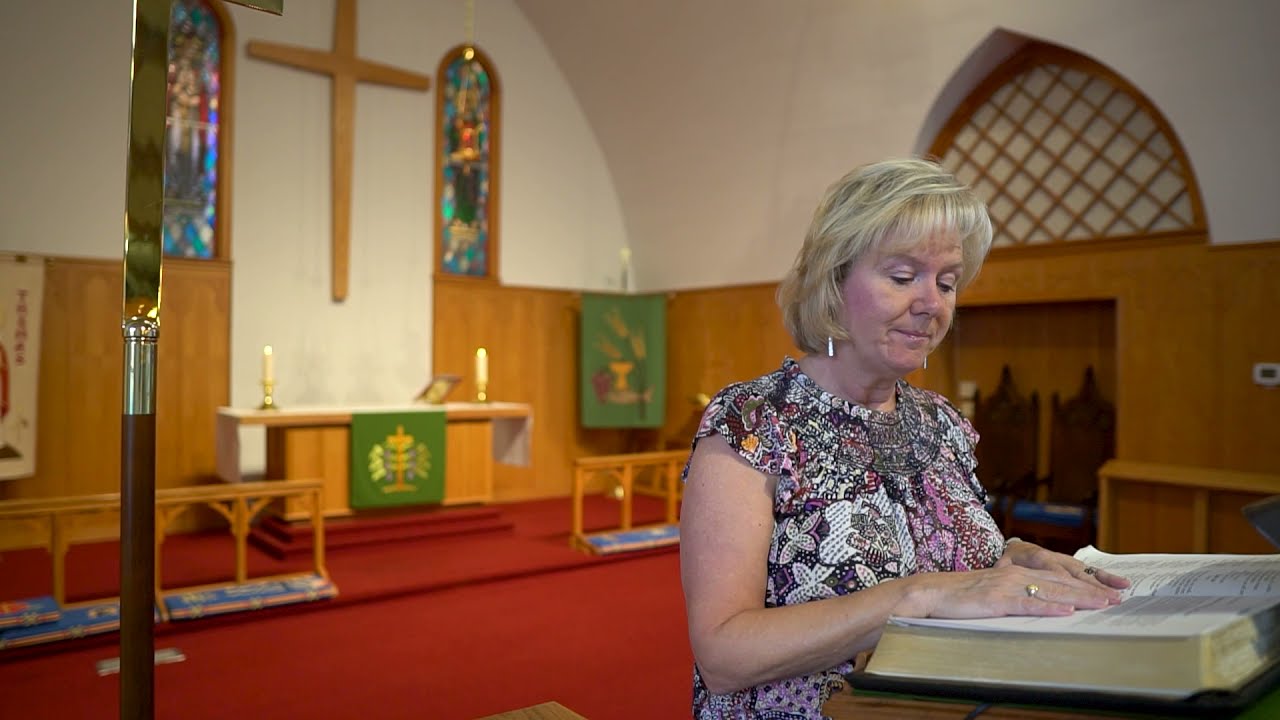In this image, a mature woman with blondish hair, likely in her 50s, stands behind a wooden pulpit in a church. She is wearing a pink, white, and black floral short-sleeve blouse and gold earrings. Both her hands rest on an open Bible, indicating she is reading from it. The church's interior features a red-carpeted stage, with a wooden cross mounted on the white wall behind her. Flanking the cross are stained-glass windows. The altar area, slightly elevated with a step up, displays a green banner and two tall candles. Additional elements include a recess with two chairs and a metal pole on the left edge of the image. The overall ambiance is typical of a church setting, with solemn decor and religious symbols.